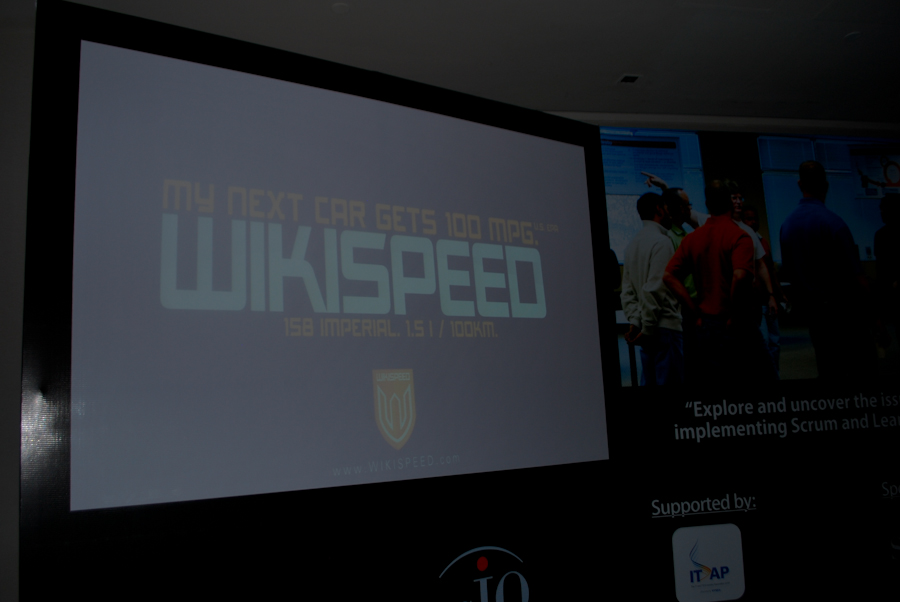The image captures a presentation in a dimly-lit room featuring a projected image on a large screen with a black border. The screen displays gray background content with prominent white text reading "WikiSpeed" across the center. Above this, in yellow or orange text, the phrase "My next car gets 100 miles per gallon" is visible, accompanied by some additional information in smaller yellow text beneath it. At the bottom-center of the screen, there's a yellow and white shield-like logo.

To the right side of the image, a banner displays a group of people gathered in a meeting room, possibly listening to a speaker. Below this banner, text includes "Supported by" with the white square logo containing the letters "I-T-A-P." The composition suggests the presentation highlights WikiSpeed's fuel-efficient vehicles and is supported by ITAP.